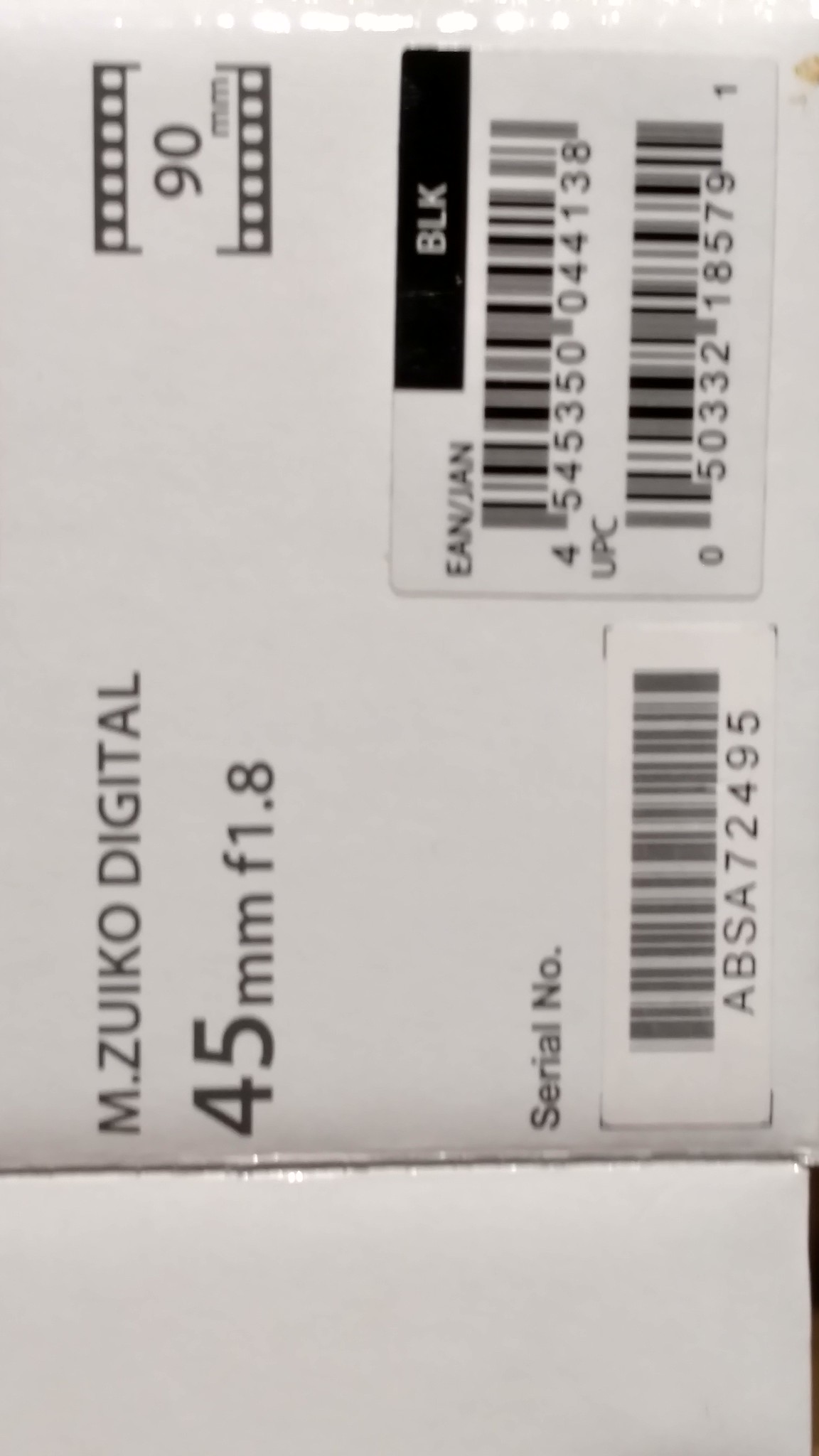The image depicts a white rectangular cardboard box or envelope with a folded-up bottom flap. The main text, oriented sideways, reads "M. Zuiko Digital 45mm F1.8" in black print at the top. Additionally, it mentions "90mm" below that and includes several printed details: a barcode labeled "UPC," another labeled "BLK EAN/JAN," and a serial number "ABSA 72495." The background is predominantly white, and there is a black label on the right side.